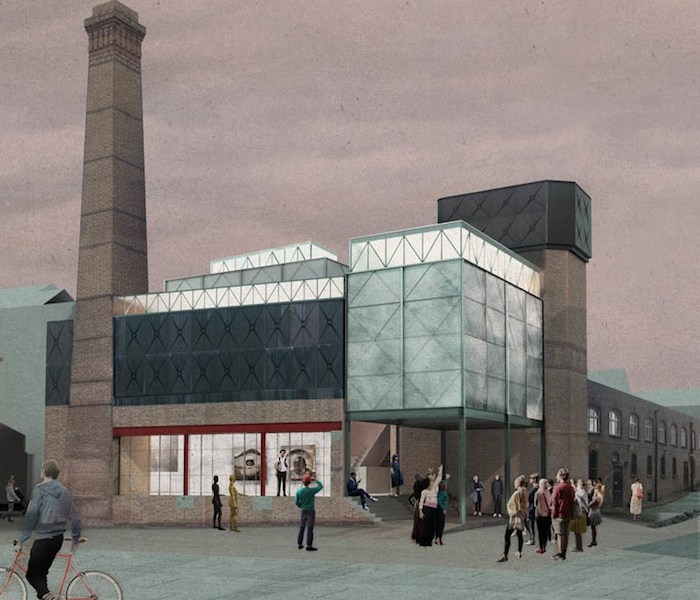The image depicts a computer-rendered painting of a 20th-century factory scene taking place at dusk. The sky is a muted grayish-pink, suggesting the approach of nighttime. The factory building is constructed of brick and incorporates numerous glass panes and steel elements within its façade. A tall brick chimney anchors the left side of the structure, while a smaller building with multiple windows and doors sits to the right. A garage or vehicle bay is discernible on the far left.

A prominent entrance with stairs features in the front, flanked by long criss-crossing beams forming windows. A small crowd of people is gathered in the courtyard, some standing on the steps and facing the building. A few individuals are scattered to the left of the scene, one of whom is wearing a hoodie and riding a red bicycle in the bottom right foreground. The detailed architecture and composition, paired with the gathered figures, evoke a sense of historical industrial life captured through digital art.